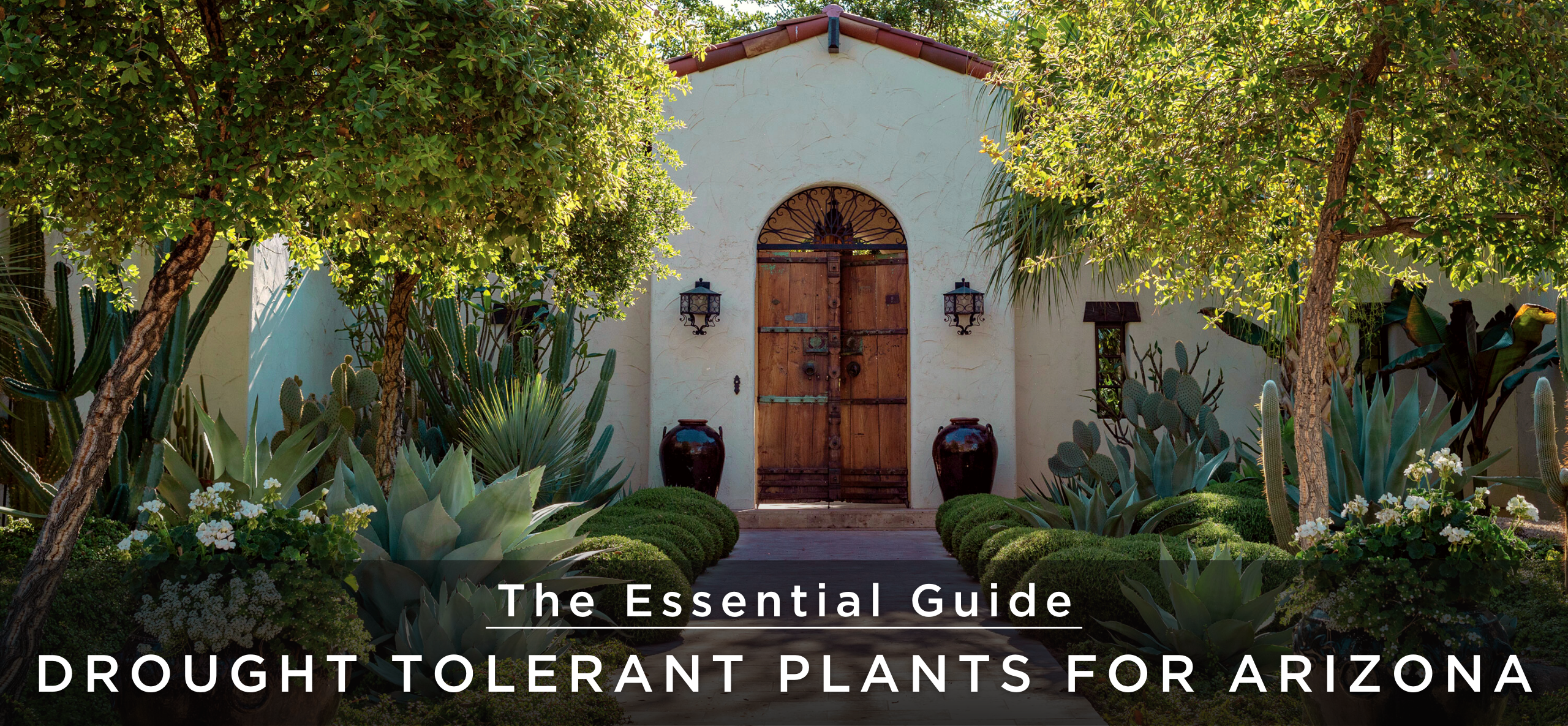The image showcases the front of a well-maintained house, dominated by a prominent, circular-topped wooden door. Flanking the door are two large black vases and two black, squarish lanterns. The walkway leading to the door is concrete, casting shadows that give it a grayish-brown hue. On either side of the walkway, a meticulously manicured garden features oval-shaped shrubs, white flowers, and various exotic plants, including cactus. To the right of the door, a statue of an eagle stands proudly. The house itself is constructed from concrete and includes a black window. Above the entrance, a camera is visible, ensuring security. The scene is bathed in sunlight, highlighting the trees and the garden's vibrancy. At the bottom of the image, a semi-transparent black bar displays text in white capital letters: "The Essential Guide – Drought-Tolerant Plants for Arizona."